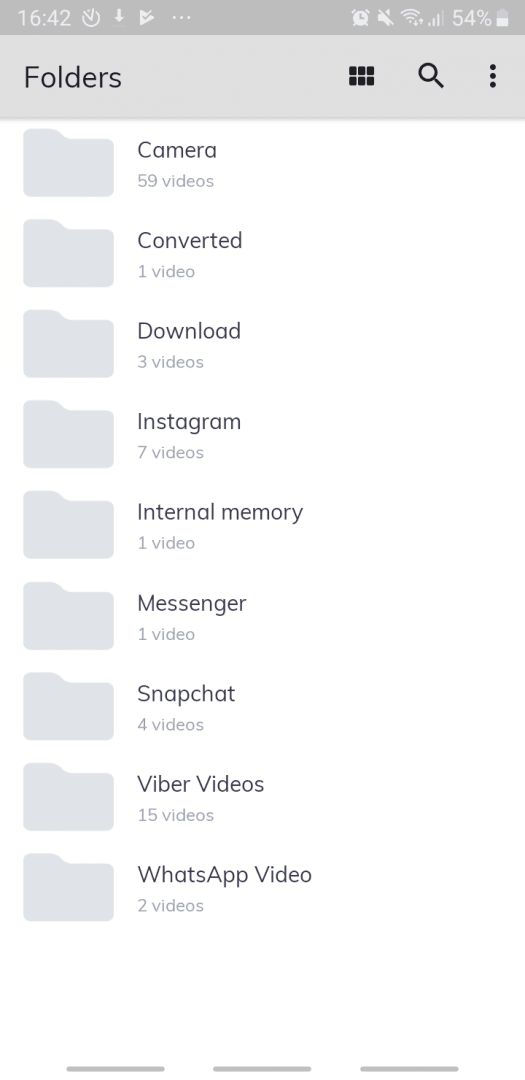The image showcases a smartphone screen displaying its various folders and organizational icons. In the upper left-hand corner, the time is clearly visible, reading 16:42, accompanied by several icons: a clock, a downward-pointing arrow, a bright-facing arrow with a checkmark in the middle, and a horizontal trio of dots. This section is presented on a gray banner. On the right side of this banner, additional symbols cluster together: an alarm clock, a mute button, a Wi-Fi signal, a cellular signal indicator, the number 54%, and a battery icon also showing 54%.

Below this darker gray banner, a wider, lighter gray banner appears with the label "Folders." This banner also includes icons for a six-square grid in black, a search magnifying glass, and a vertical trio of dots. Proceeding downwards, the images transition into gray folder icons, each with associated black text detailing the contents of each folder. These include:

- Camera: 59 videos
- Converted: 1 video
- Download: 3 videos
- Instagram: 7 videos
- Internal Memory: 1 video
- Messenger: 1 video
- Snapchat: 4 videos
- Viber Videos: 15 videos
- WhatsApp Video: 2 videos

At the bottom of the screen, three long, horizontal gray lines are aligned parallel to the rest of the displayed information, providing a subtle visual guide.